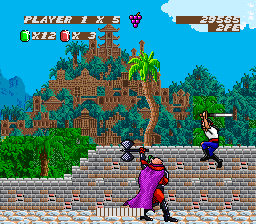This screenshot captures a scene from an older-style video game. The player character, viewed from behind, is adorned in a flowing cape and sturdy black boots, wielding a double-sided axe in their left hand. The character is in mid-swing, suggesting an imminent attack. To the right, an NPC is suspended in the air with a sword poised dramatically overhead, seemingly engaged in combat. The background features a wooden structure and a wall, contributing to the game's rustic, immersive setting.